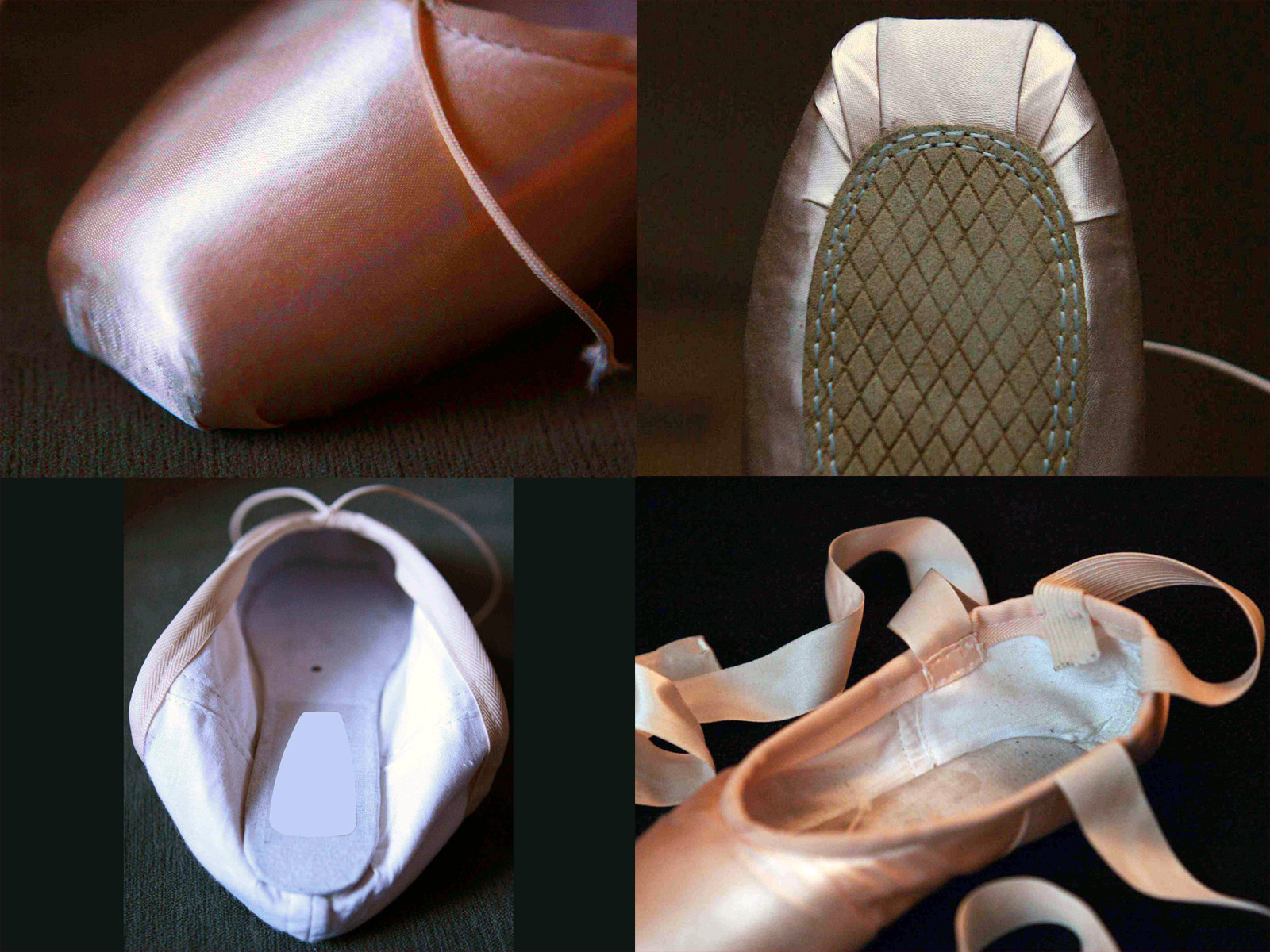The image showcases a detailed collage of four close-up, color photographs of pink ballet slippers, arranged in quadrants over a wooden surface with black background. In the upper left quadrant, there is a close-up of a ballet slipper's toe, highlighting its delicate pink fabric and brownish ribbons. Moving to the upper right quadrant, the image captures the bottom front half of a ballet slipper, displaying the pink satin fabric, intricate cross-hatch stitching, and a view of the foot padding. The lower left quadrant offers an inside look from the back of the slipper, exposing the gray sole and the white lining, with openings on either side of the shoe. Finally, the lower right quadrant provides a glimpse of the back of the slipper, showing the peach-like exterior, the sewn-in straps, and an open view into its interior. Throughout all images, the ballet slippers rest on a textured wooden surface while maintaining a black background, emphasizing the delicate details and craftsmanship of the ballet footwear.